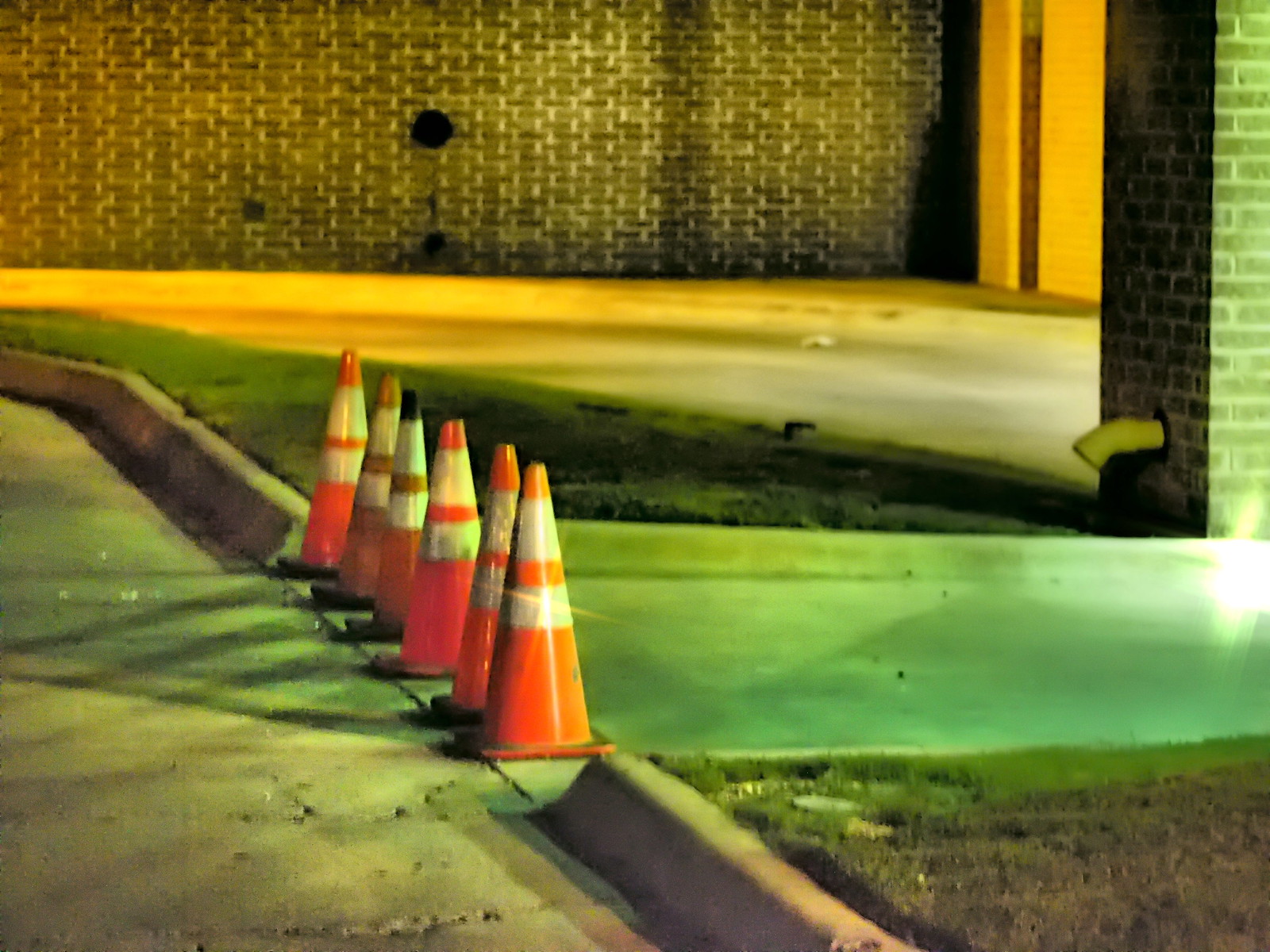The image depicts a section of a parking garage with a driveway leading into it, flanked by a large brown brick wall with some black circles in the middle. The entryway to the parking garage is illuminated with a yellow light. In the foreground, six orange traffic cones with white stripes are arranged in a row, blocking off a sloped walkway that veers to the right. To the left of the walkway, there is a pillar, and on both sides of the walkway, there are grassy medians. The cones are positioned on the freshly tarred or cemented pavement, likely to prevent people from walking or driving on the still-setting surface.